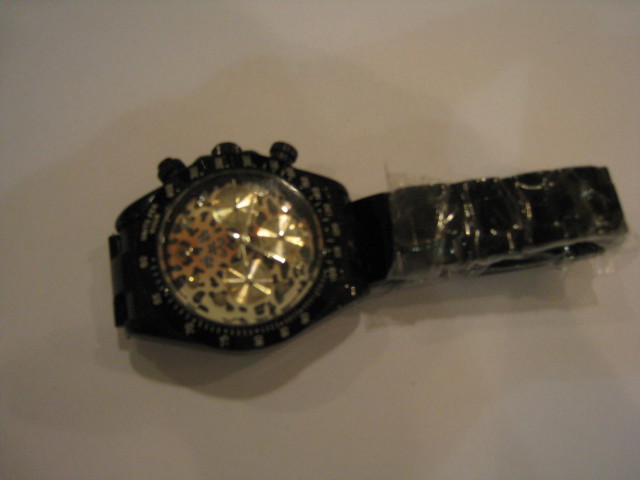This dimly-lit and slightly blurry photograph captures a wristwatch resting on a white surface. The watch face, positioned on the left side of the image, features a distinctive cheetah print design and houses three smaller sub-dials within. The outer edge of the face is adorned with numerical markers, while the inner portion has none. Gold hour and minute hands elegantly sweep across the watch face. The solid black wristband, extending to the right side, appears to have a piece of protective plastic still attached. The overall composition of the image, coupled with the intricate details of the timepiece, draws attention to its unique and stylish design.